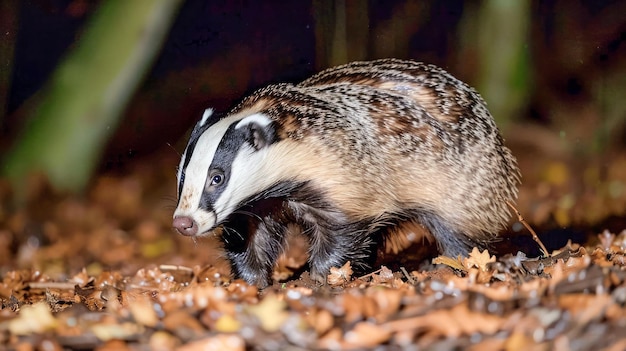The photograph captures a small, four-legged creature, possibly a badger, standing on the ground in an outdoor setting. The animal has a white face with a long snout and a pinkish-tan nose. It features distinct black stripes running from the nose, across the eyes, and back over the ears. The fur on its head is brushed back and is cream-colored, while the rest of the body displays a patchy mix of browns, grays, creamy colors, and whites. The legs are short and covered in dark, possibly black fur. The badger is positioned facing the left side of the image, where a soft light source is illuminating it from the center-left. The background is out of focus, revealing blurry green sticks or sprigs, and the foreground consists of various shades of brown with crushed foliage and wet leaves, indicating a moist environment. The secluded lighting suggests an effort to avoid startling the creature.